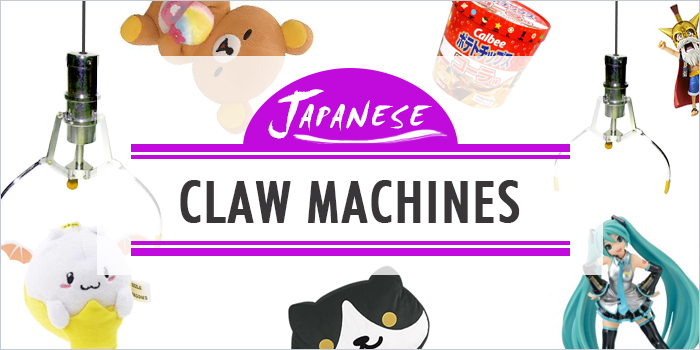The image is a detailed advertisement for Japanese claw machines, commonly found in modern settings like boardwalks, carnivals, and fairs. At the center, there's a brand logo resembling a purple sunset with the word "Japanese" overlaid on it, and a transparent background. The scene features a variety of prizes and characters that one might find inside such machines. 

Dominating the scene is a plushie anime superheroine with long greenish-blue hair, over whom a claw hovers, poised to grab her. Directly below this claw mechanism, another claw descends on a small, white animal-like figure. To the side, an older character with a white beard and red cape adds a sense of variety and intrigue. In the middle, on the bottom, sits a black and white kitty cat plushie, surrounded by additional prizes. 

At the top of the image, a tan teddy bear holding what looks like a softball is showcased, next to a reddish container that likely holds some sort of treat, perhaps cotton candy. The overall illustration places a heavy emphasis on these modern and vibrant figures against a clean white background, making all details easily identifiable and appealing. 

The stylized nature of the advertisement, combined with its vivid depiction of the claw mechanisms and eclectic mix of Japanese popular culture mascots, snacks, and anime figures, highlights the allure and excitement of these captivating machines.